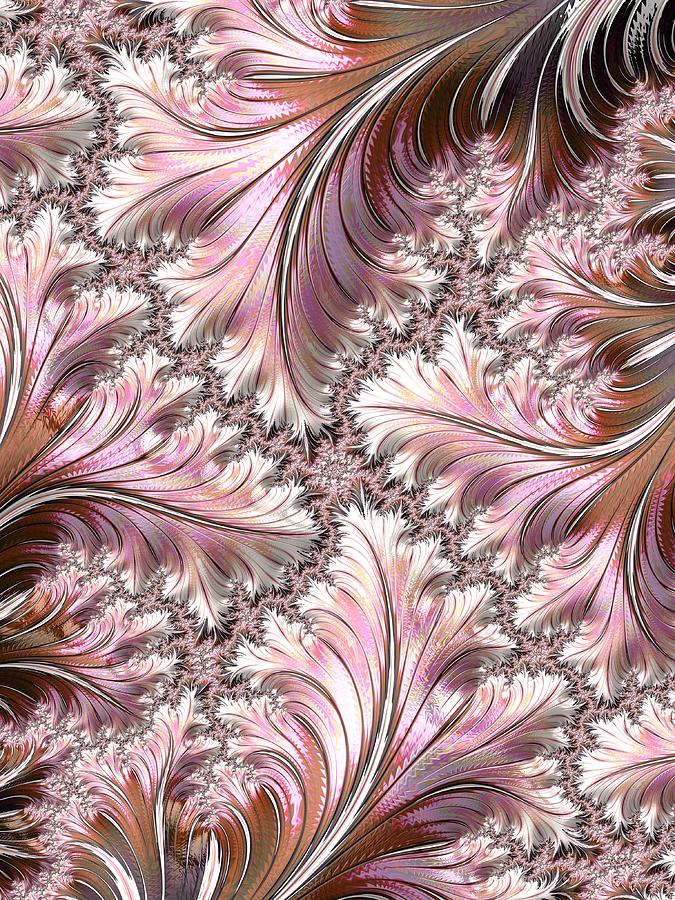The image is an intricate and colorful illustration of large, wispy feathers fanning out from the center of a white background, almost like a fractal pattern. The feathers showcase a gradient of colors, starting with deeper shades such as browns, purples, and dark reds at their bases, and transitioning into lighter hues of pinks, yellows, and white tips. Among the mass of feathers, four particularly prominent ones stand out, including one emerging from the top right corner and extending downwards. Pink fuzz or lines intricately separate the feathers, adding to the softness and gentle nature of the artwork. Despite the multitude of feathers—approximately seven or eight—the palette remains harmonious, with most feathers sharing similar shades, though one in the upper right corner exhibits more black. The overall aesthetic evokes a sense of delicate beauty, reminiscent of ostrich plumes, wallpaper, or even finely detailed clothing fabric.